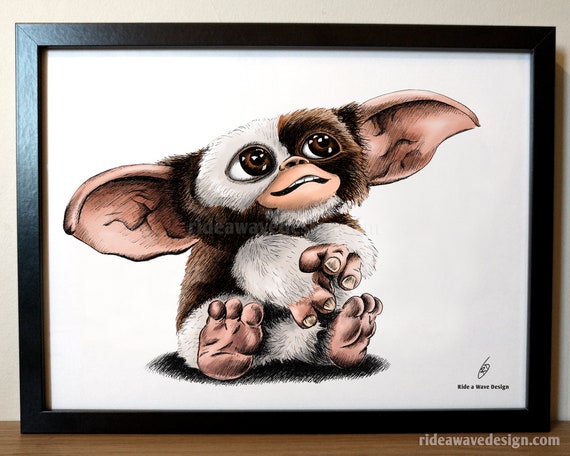In this photograph, a framed drawing of the Mogwai Gizmo from the film Gremlins is prominently displayed on a wooden table against a white wall. The black frame encloses the detailed artwork on a white background, showcasing Gizmo with large floppy ears and fur that alternates between white and brown. Notably, Gizmo's face features a white spot over his left eye, with the other side being brown. His expressive, large brown eyes gaze upward towards the top right corner, enhancing his endearing and playful demeanor. Gizmo's fur-covered body extends to all areas except his distinctly human-like hands and feet. The drawing includes the text "ridewavedesign" in the bottom right corner as well as a semi-transparent watermark in the center, accompanied by a URL in white semi-transparent text reading "ridewavedesign.com." The detailed craftsmanship of the drawing highlights Gizmo's charming features and nostalgic significance as the benevolent character from the beloved movie.